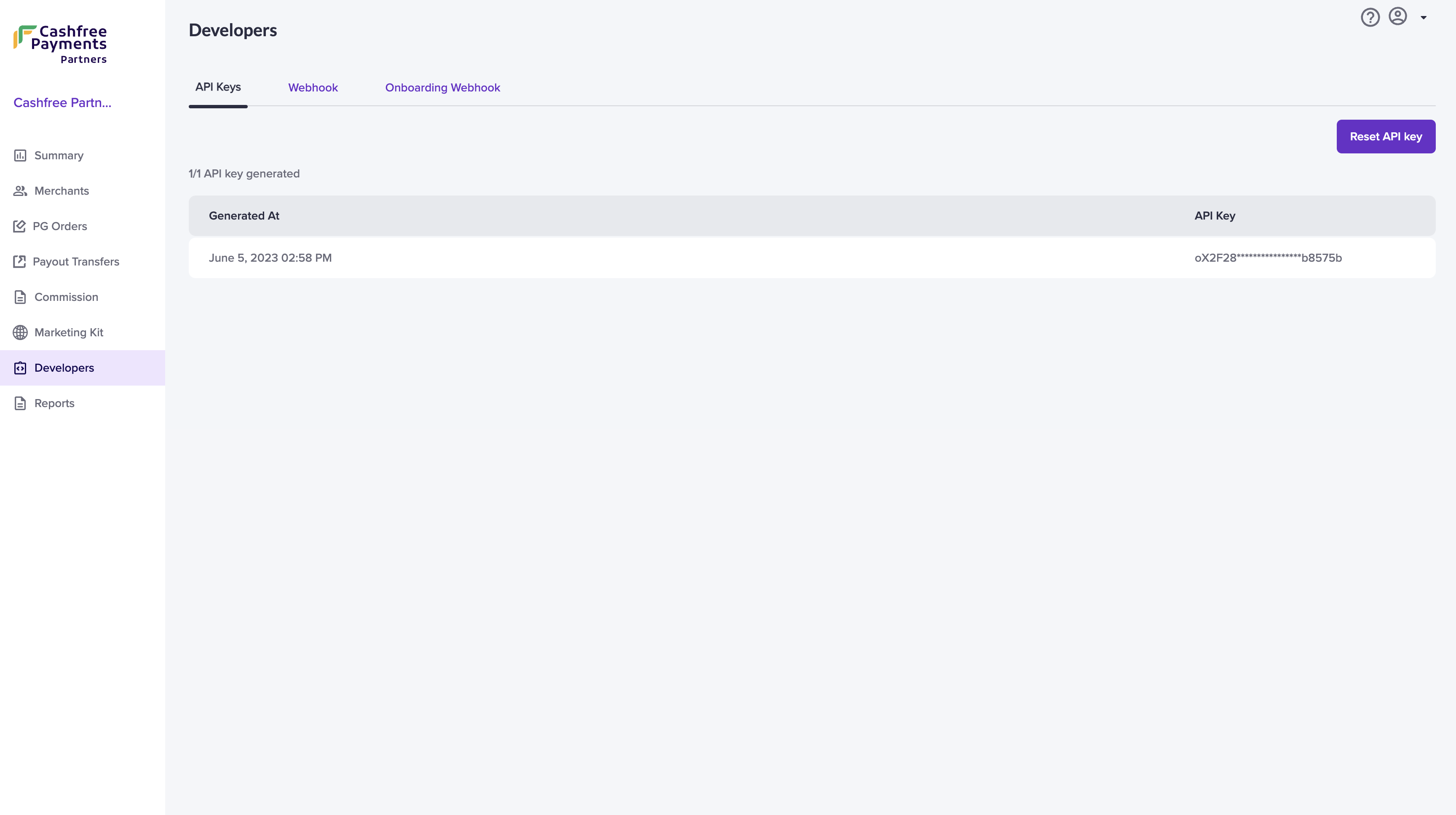In the image, the top left corner prominently displays the brand name "Cash Free Payments Partners". Below the brand name, there's a geometric icon featuring an intersecting green and yellow line. Underneath, it displays the URL "CashFreePayments.paypartn.com", followed by a set of menu items: Summary, Merchants, PG Orders, Payout, Transfers, Commission, Marketing Kit, Developers, and Reports all listed in grey text.

On the far top left, it highlights "Developers" in black text. Directly below, there are the sub-sections "API Keys" and "Webhook". The main section is focused on "Homeboard and Webbook", detailing a specific entry: "API Key Generated, June 5th, 2023, 2:50 PM" in grey text. Further indicating "Date Key" is listed below this section. 

Above this section, there's a prominent purple, hyperlinked box with the white text "Request API Key". At the top right corner of the image, there's a question mark icon, a gray person account icon, and a dropdown menu. The majority of the image background is grey. The "API Keys" section is highlighted with a slightly darker purple and yellow hue and is underlined, indicating it is the selected option.